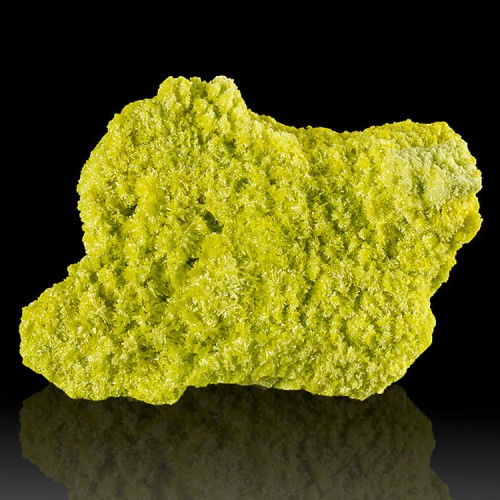The image features a close-up of an irregularly-shaped, light olive green object resembling a porous rock or sponge. Despite its spongy appearance, the object appears more solid than soft. It has a rough and craggy texture, with small fuzzy growths resembling white specks scattered throughout its surface. The object is rectangular but slightly uneven, with some points around its edges, and it is positioned such that the top part is slightly offset to the right of the bottom part. This unusual green object rests on a reflective surface, mirroring its form in a lighter hue. The entire scene is set against a stark black background, providing sharp contrast and making the object appear almost illuminated or glowing, though no size reference is provided.